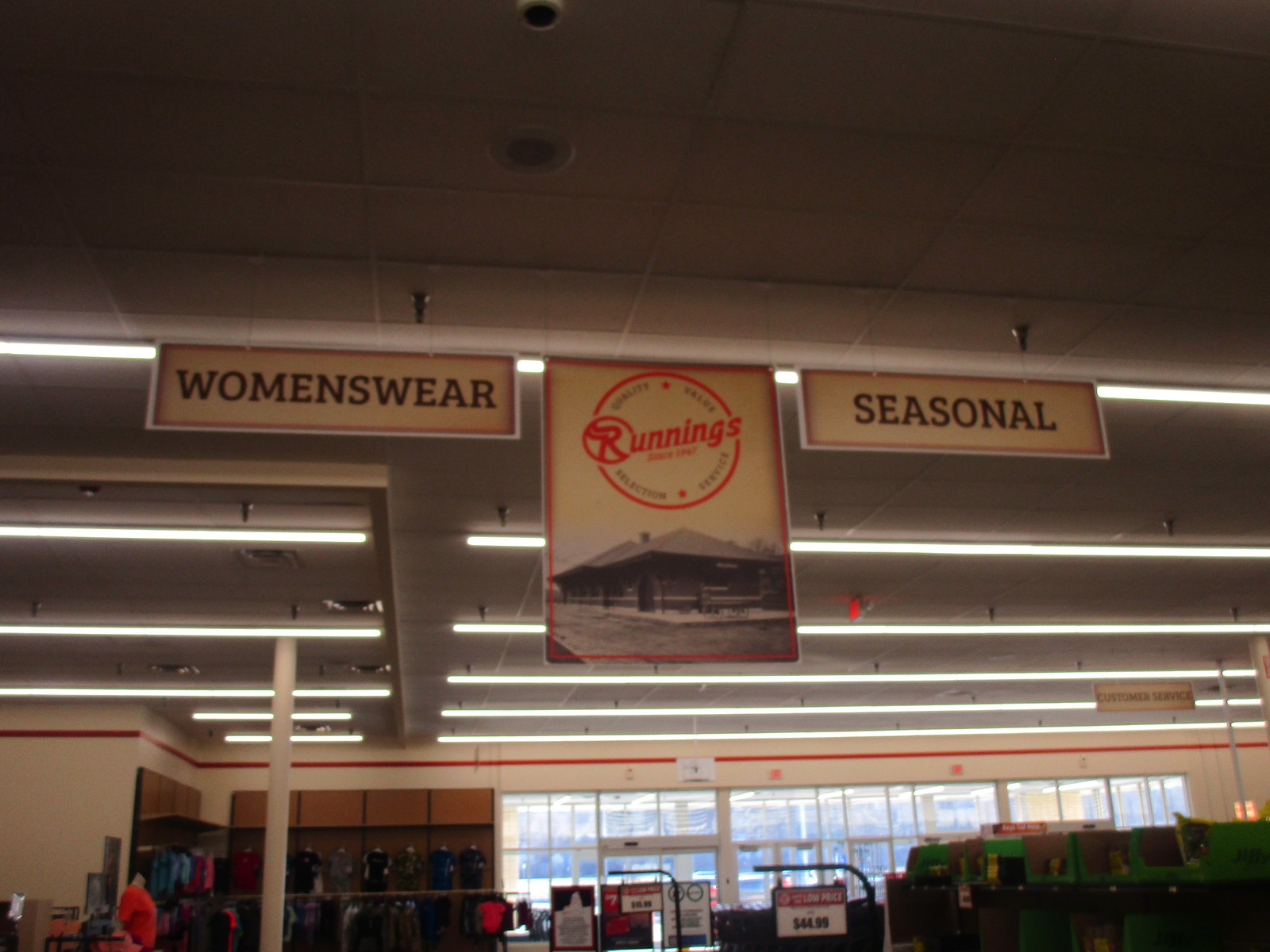An interior shot of a clothing store, captured from a low angle that emphasizes the ceiling. Dominating the center of the image is a hanging sign featuring the "Runnings" logo in bold red text encased in a red circle. Directly beneath this logo hangs a black and white photograph of a single-story building. Flanking the central sign, two rectangular signs with a yellowish tint are visible, reading "WOMEN'S WEAR" and "SEASONAL" in black capital letters. The ceiling above showcases an industrial or school-style design with removable panels and long fluorescent lights. A striking red line runs along the upper wall of the store, adding a touch of color to the otherwise muted surroundings. In the bottom right corner, some merchandise is partially visible, while the bottom left corner reveals a glimpse of clothing.